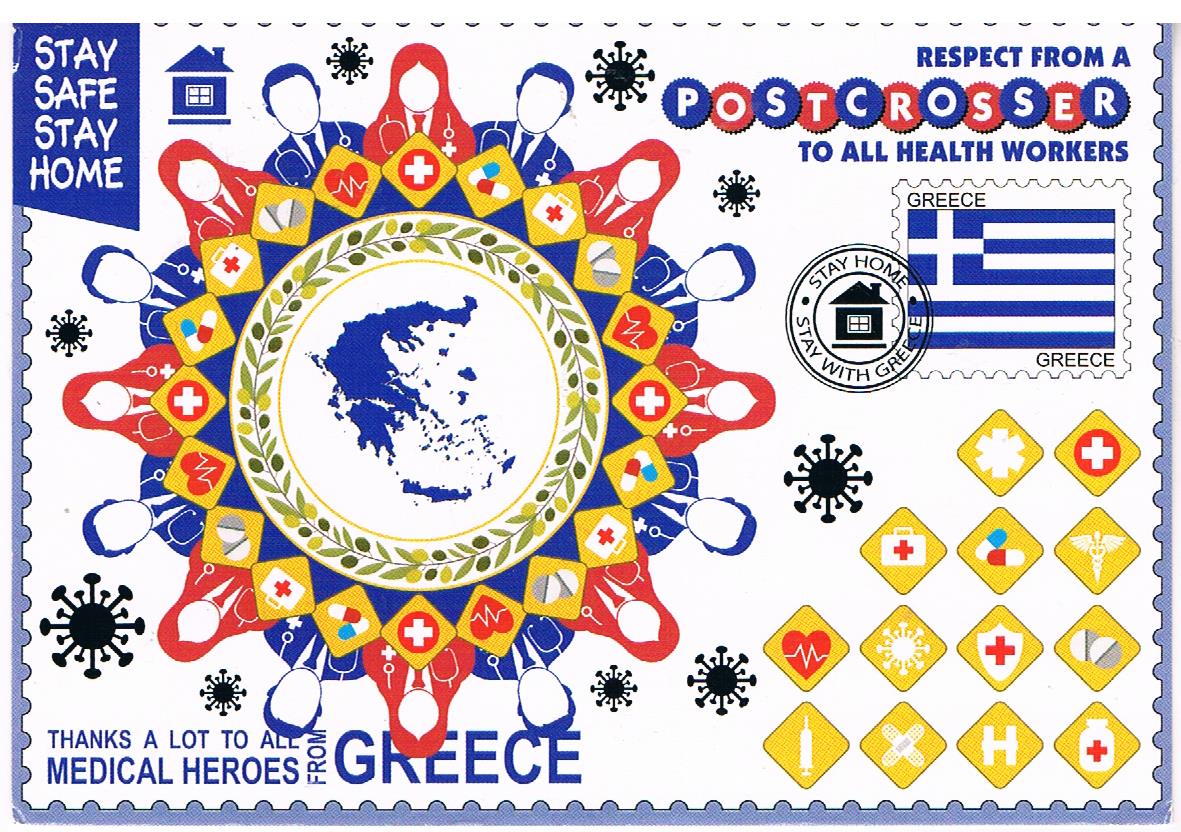This intricate and colorful postcard-like image, possibly an enlarged commemorative stamp, honors healthcare providers during the pandemic. Dominated by hues of blue, red, white, yellow, light blue, and gray, it features a central motif of a circular table surrounded by 16 alternating red and blue silhouettes of medical professionals wearing stethoscopes. The figures, faceless and split evenly by gender, encircle an artistic depiction of the Greek Isles set within a white background, itself bordered by foliage and a band of blue.

Adorning the upper left corner, the text "Stay Safe, Stay Home" is accompanied by a small home icon, while the bottom left declares in blue uppercase letters, "Thanks a lot to all medical heroes from Greece." The upper right corner emphasizes, "Respect from a Post-Crosser to all health workers," with each letter of 'Post-Crosser' encased in alternating blue and red circles. Spread throughout the white background, black coronavirus icons are interspersed with 13 yellow diamond-shaped symbols featuring various medical emblems.

Framing this bustling design is a serrated edge, resembling that of a postage stamp, suggesting its commemorative nature. Just inside this border, another serrated frame surrounds the word "Greece" alongside the Greek flag in blue and white, overlaid with the message "Stay Home, Stay with Greece" encircling a home symbol resembling a postmark. This heartfelt tribute, brimming with gratitude, reflects the global sentiment of appreciation for medical heroes during the pandemic.